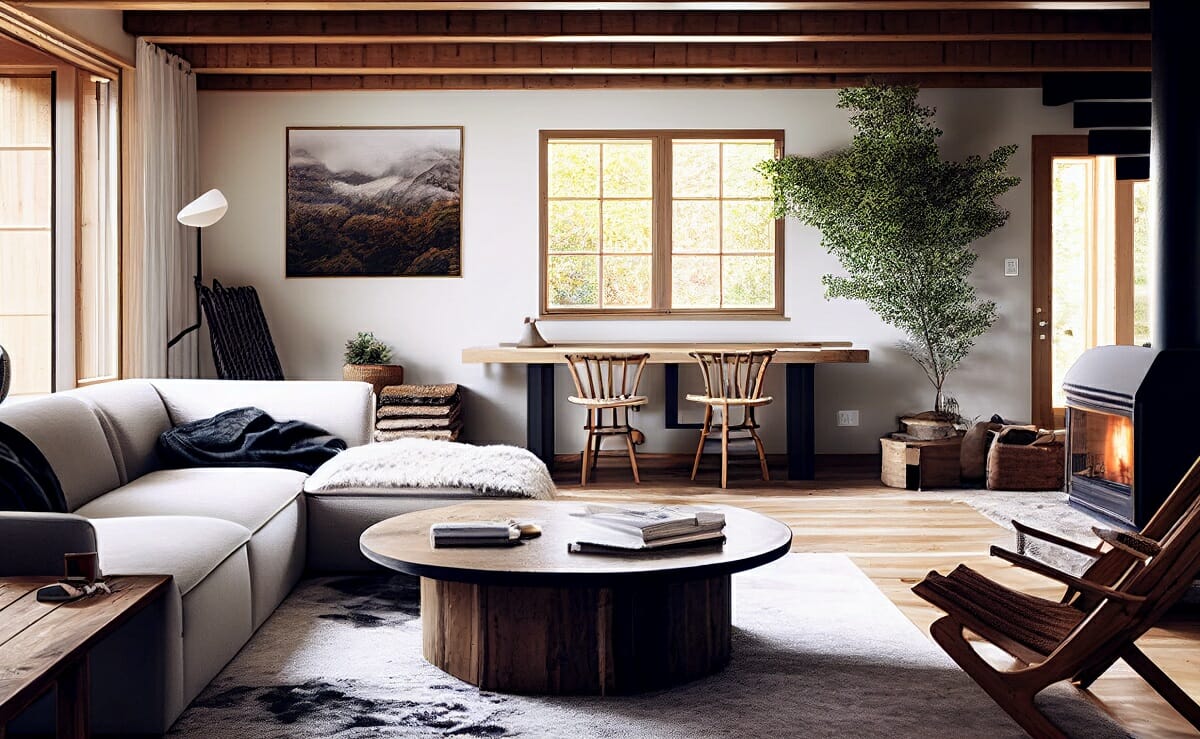This photo, taken during the day, captures a cozy, well-furnished living room in horizontal landscape orientation. The focal point on the right side of the room is a black metal fireplace with a visible flame and extending chimney. Next to it, a mid-century modern wooden reclined chair sits in the bottom right corner. In front of the chair, a round wooden coffee table with books rests on a black and white rug covering the wooden floor. Occupying the left side, a cream-colored couch adorned with a black throw blanket sits adjacent to an ottoman covered by a white blanket.

To the middle right, a window framed in wood casts natural light into the space. Adjacent to this window is a brown bar-type table with black legs accompanied by two brown chairs. On the wall above this setup, a six-paned double glass window adds a touch of classic elegance. Nearby, beneath another window, sits a landscape painting flanked by shelving and a potted plant.

The room also features an artificial—possibly real—tree in a brown basket, adding a fresh green touch among brown pots and baskets placed nearby. The ceiling displays exposed rafters, enhancing the rustic charm. The left side of the room includes curtains, more windows behind the sofa, and a reading lamp over what appears to be another chair. This thoughtful arrangement creates a warm, inviting atmosphere, blending modern and rustic elements seamlessly.